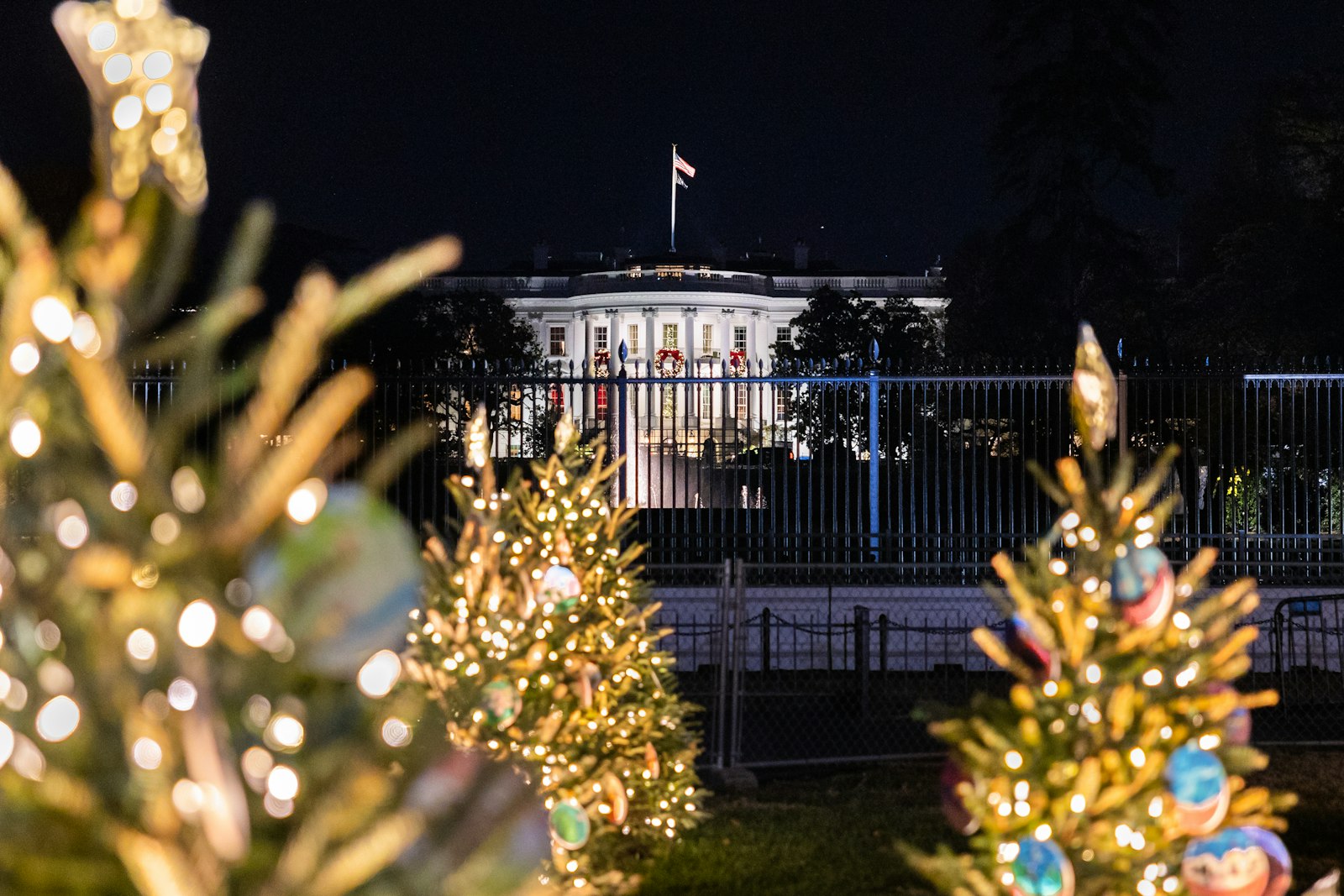This nighttime photograph captures the White House adorned for Christmas against a pitch-black sky. The iconic building, set in the center of the frame, features classical-style pillars leading up to a rounded roof, crowned with two American flags flying to the right. Silhouetted trees flank either side of the White House, adding a natural touch to the scene, while an iron palisade fence with sharp points separates the grounds from the immediate surroundings. In front of this, a chain-link fence lines a closer road. The foreground is dominated by festive Christmas trees, slightly blurred but detailed enough to show their green and gold lit branches, white dotted lights, and blue and red baubles. A large, close Christmas tree stands prominently to the left, with two more in succession creating a festive corridor, and a lone tree appears on the right side of the frame. This festive arrangement enhances the majestic appearance of the White House, emphasizing the holiday spirit amidst the stately ambiance.